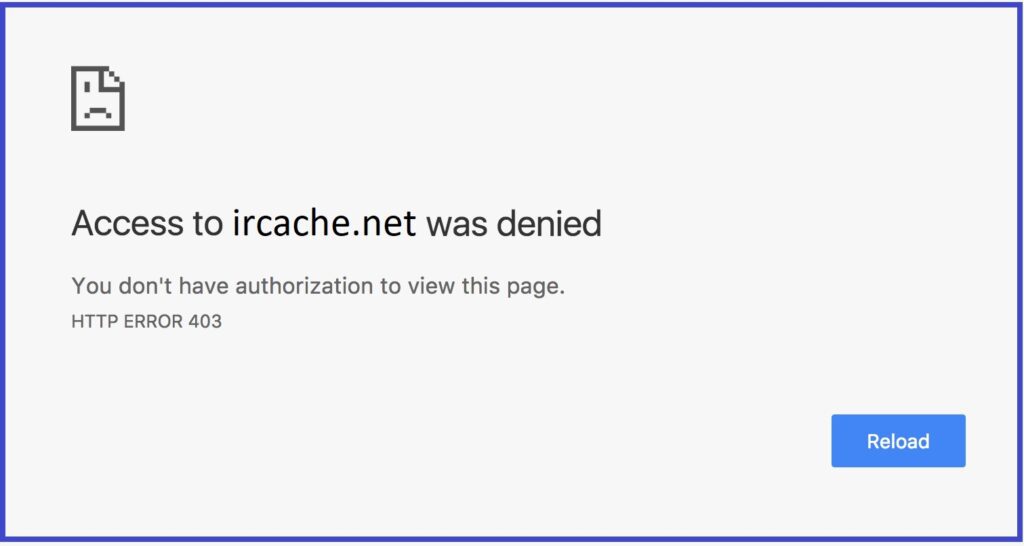The image depicts an error message with a white box that has a thin purple frame. The box is oriented such that its width is greater than its height. Inside the box, towards the bottom right corner, there is a blue "Reload" button with white text, positioned approximately three tab spaces from the bottom and two from the right side. At the upper left corner of the box, there is an icon of a dog-eared page with a frown face. The message in the box reads, "Access to IRCache.net was denied," followed by the HTTP error code 403. This clear and concise yet detailed caption captures the essential elements of the image.